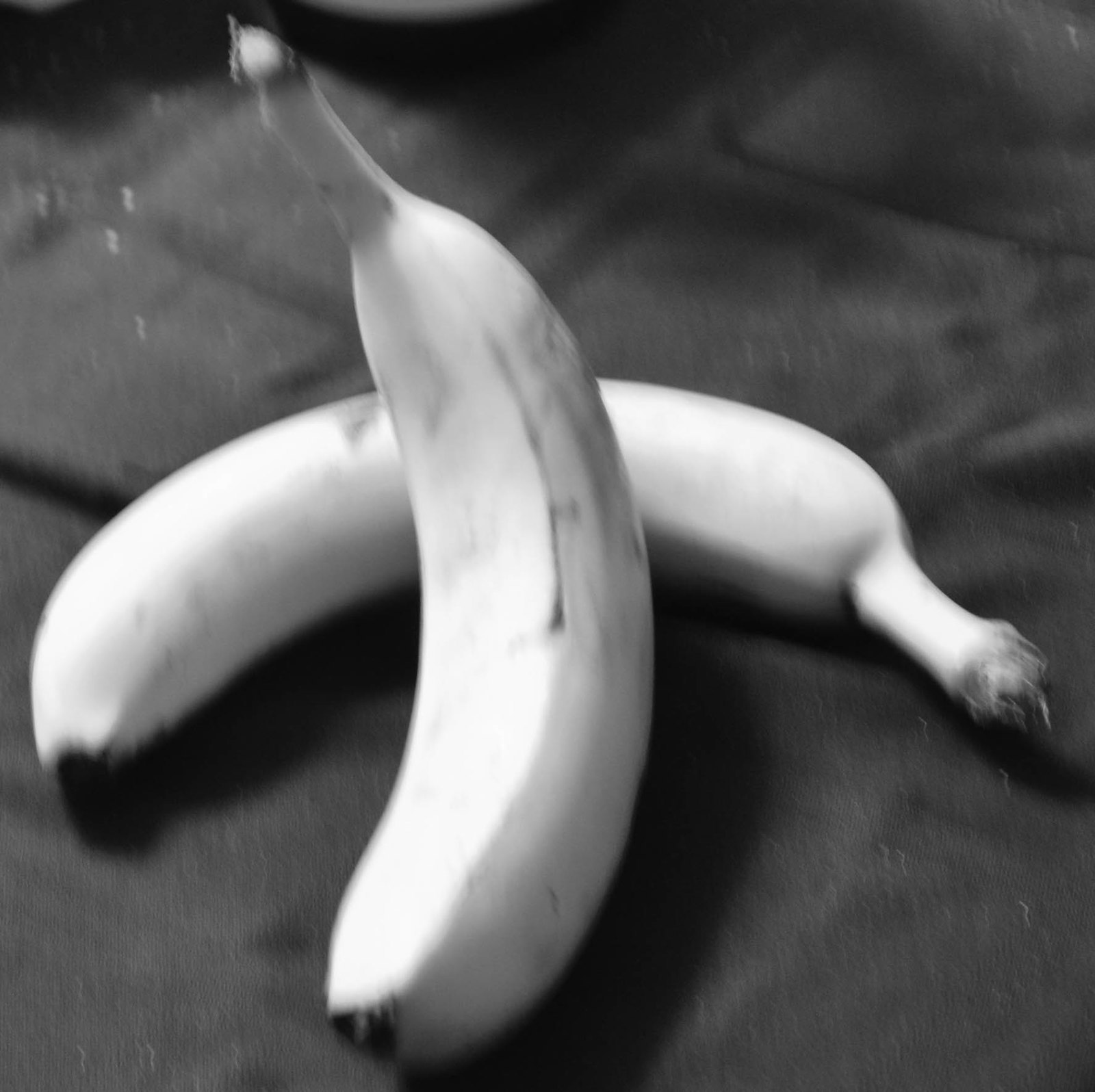In this black and white photograph, two bananas are presented against a dark grey fabric backdrop. The fabric appears to be draped over an uneven surface, as evident by several square-shaped protrusions on the left, numbering two or three, and additional indentations moving towards the center and right. 

The first banana lies horizontally with its stem on the left and the tip on the right. Its stem shows slight fraying, resembling tiny strands of hair. The second banana stands upright in the center of the image. Its long stem extends towards the top and slightly leans to the left, with the bottom stub also slightly tilting to the left. This upright banana features a black line that runs halfway up its length, gradually fading, and exhibits a small area of brownish bruising on its right side.